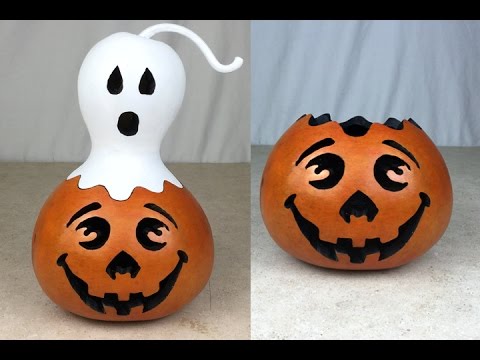The image features two smooth, brownish-orange jack-o'-lantern decorations set against different backgrounds, emphasizing their Halloween theme. Both jack-o'-lanterns have a painted smile with teeth, triangular noses, and circular eyes with eyebrows. The one on the left is in front of a gray backdrop and is topped with a white ghost figurine, whose bottom scallops seamlessly fit the jack-o'-lantern's scalloped top. The ghost has an oval face with an "O" expression and a single strand of hair. The jack-o'-lantern on the right, placed against a light blue background, lacks the ghost and showcases its open, scalloped top. Both jack-o'-lanterns are likely made of metal or plastic and appear to be designed for Halloween decorations, possibly shown in a catalog-style photograph.